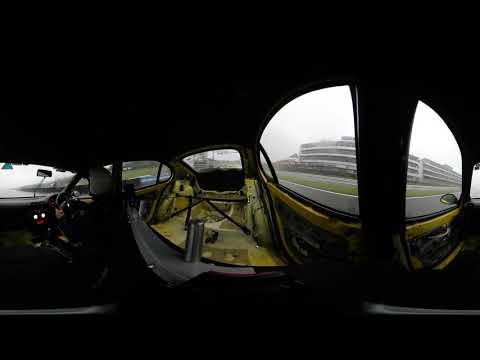This image captures the inside of a race car in a derelict state, taken with a warped, panoramic effect that distorts the interior. The stripped-down yellow metal frame is prominently visible, with the driver's seat occupied by a race car driver wearing a white helmet and a black racing suit. The driver sits on the left side, hands on the steering wheel, with the black roll bars extending from the back of the car to the front windshield. The dashboard has two illuminated dials, likely a speedometer and tachometer, alongside a gear shift on the left side of the console. Outside the car's windows, there's overcast, foggy weather and a large, white, corporate-style building resembling a hospital. The street appears empty with no other vehicles in sight.